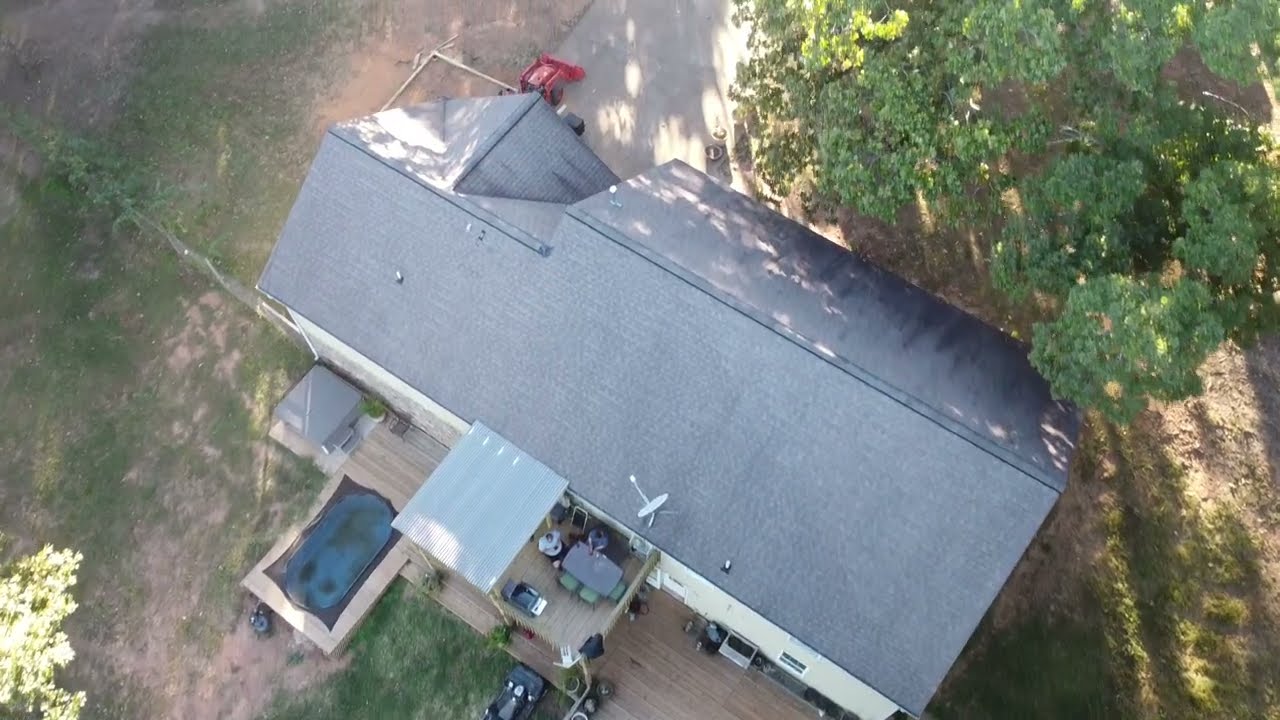This aerial photograph, taken during the daytime, presents a detailed view of a residential home and its surrounding area. The house features a light grey, triangular-shaped roof without a chimney, but with an attached satellite dish. The driveway at the front of the house is white and has a red piece of equipment in it. The backyard includes a noticeable awning, a large outdoor dining table with six chairs—two of which are occupied by individuals wearing blue and white shirts—a grill, and a possibly a jacuzzi or hot tub. The porch appears to be made of wood. The ground around the house consists of both green grass and patches of brown soil, with some sparse greenery and a couple of trees, one positioned at the front right side and another in the backyard on the left side.